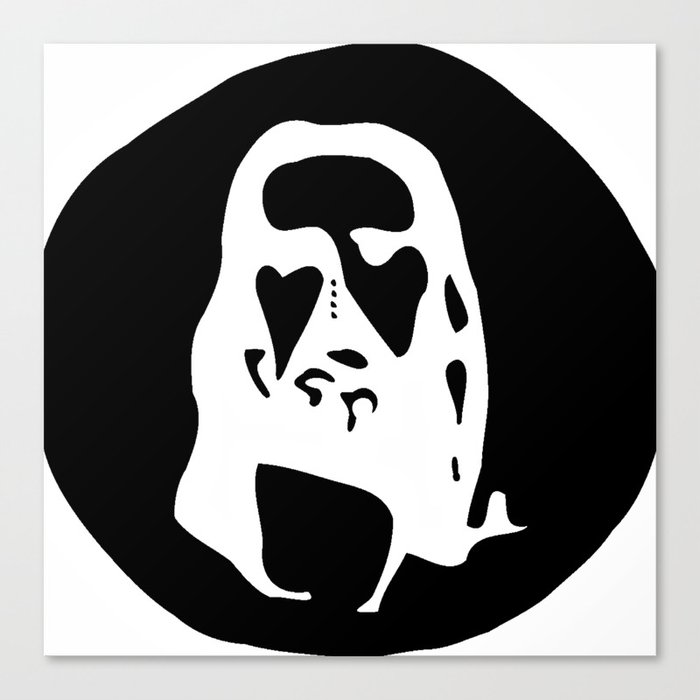The artwork in question is an intricate black-and-white illustration set against a solid black background. This abstract image primarily features an enigmatic white face or head shape, which some may interpret as having a resemblance to the face of Jesus or even Chewbacca due to its long hair and serene, somewhat indistinct expression. The eyes are particularly notable, with one resembling a heart shape and the other embodying a more ambiguous, perhaps thought-provoking form. The depiction includes various details, such as a series of dots where the nose might be, a black outline suggesting the mouth, and additional black areas that represent the forehead and parts of the hair, which appears to cascade to shoulder length and tapers off to the right side. The piece exudes a sense of fluidity and transformation as different viewers might see different figures or symbols the longer they look. It is presented on what seems to be a textured or canvas-like material, bordered by a gray fringe, adding to its tactile, paper-cutout aesthetic.